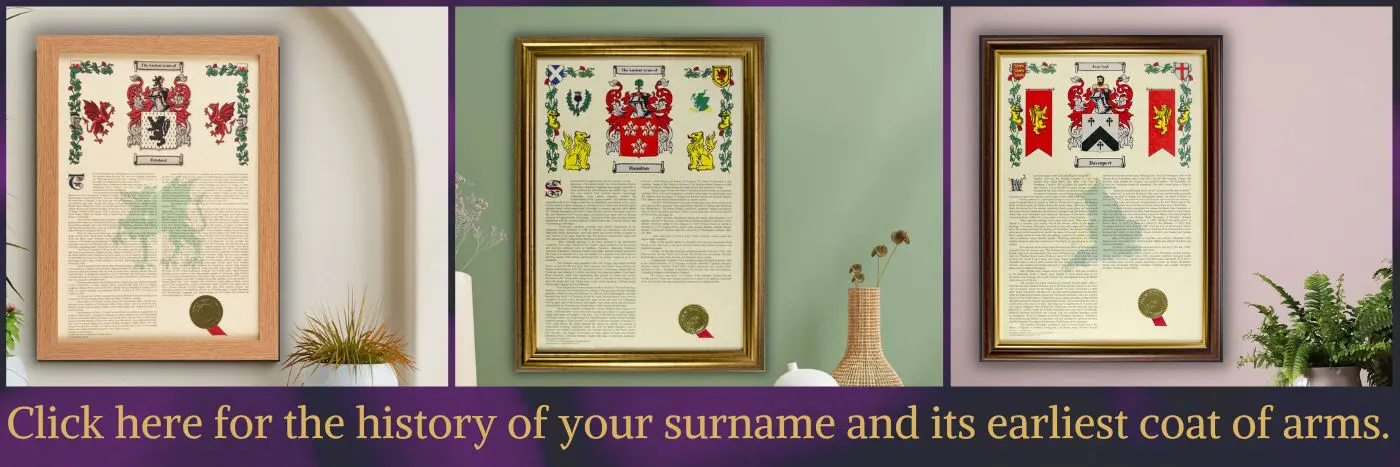The image is a three-part photograph with each section displaying a distinct framed illustration of a coat of arms, accompanied by large text columns underneath. These three pictures are aligned horizontally, separated by a purple border, and share a common text banner at the bottom that reads, "Click here for the history of your surname and its earliest coat of arms," written in yellow letters.

### Detailed Description:
- **Framing and Backgrounds**:
  - **Left Image**: Features a coat of arms within a wooden brown frame, set against a white wall. The framed illustration resides in an alcove with a white planter containing small, spiky leaves in the bottom right corner.
  - **Center Image**: Displays a golden-framed coat of arms against a mint green backdrop. A wicker planter filled with clover-like leaves sits in the bottom right-hand corner.
  - **Right Image**: Shows a darker brown framed coat of arms against a lavender-colored wall. A white planter with fern-like leaves is positioned in the bottom right corner of this section.
  
- **Illustrations and Descriptions**:
  - Each framed illustration centrally features a distinct coat of arms:
    - **Left Image**: A white background with two phoenix-like birds in red on either side.
    - **Center Image**: A white background with a yellow winged lion on either side.
    - **Right Image**: A white background with red banners displaying yellow lions reared up with their paws extended forward.
  - Bordering the illustrations on the top left and right are green leaves, providing a decorative element.
  - Beneath each image, there are several lines of black text detailing the history of the respective surname and its coat of arms.

The unified theme across these panels suggests an advertisement for a website selling personalized family crest decorations, emphasizing the historical and heraldic significance of different surnames.